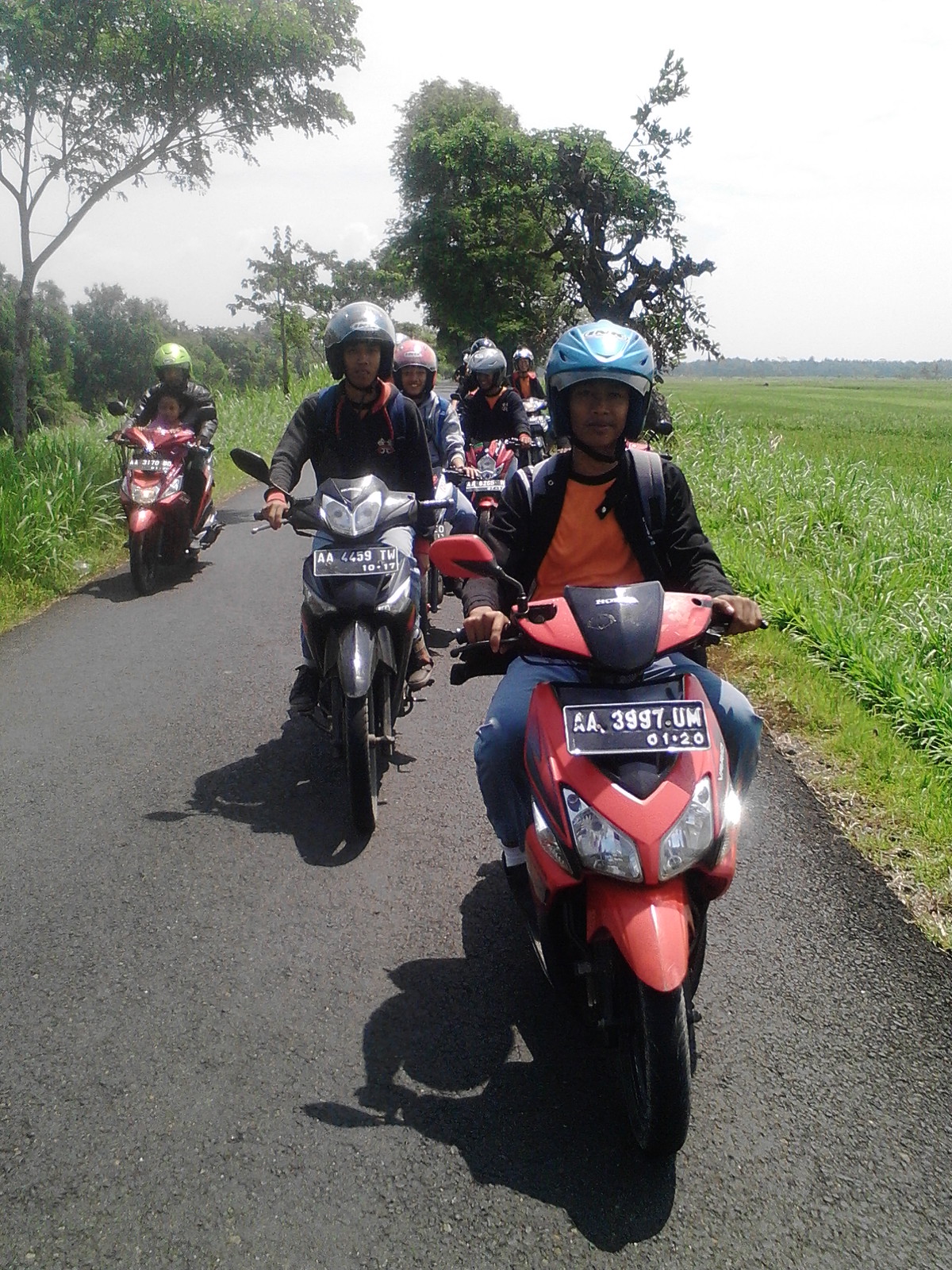This photograph captures a group of six motorcyclists riding mopeds or motorbikes on a black asphalt road, heading directly towards the camera. The riders are spread across the frame with greenery on both sides of the road, consisting of grass and shrubbery. On the left side of the image, a prominent tall tree stands, with additional trees visible in the background, indicating it's daytime due to the bright sky.

The lead rider, closest to the camera, is on a red bike with black accents and a license plate reading AA-3997-UM-01-20. This person is equipped with a blue helmet, an orange shirt, denim pants, and a black jacket. The attire of other riders also includes helmets, all black except for the rider on the far left who sports a yellow helmet, also riding a red bike.

Although the environment suggests a rural or possibly jungle-like setting, the activity clearly portrays a close-knit group enjoying a shared journey. The dynamic formation, complemented by variations in motorcycle colors and the distinct attire of the riders, adds a vivid, adventurous quality to the image.